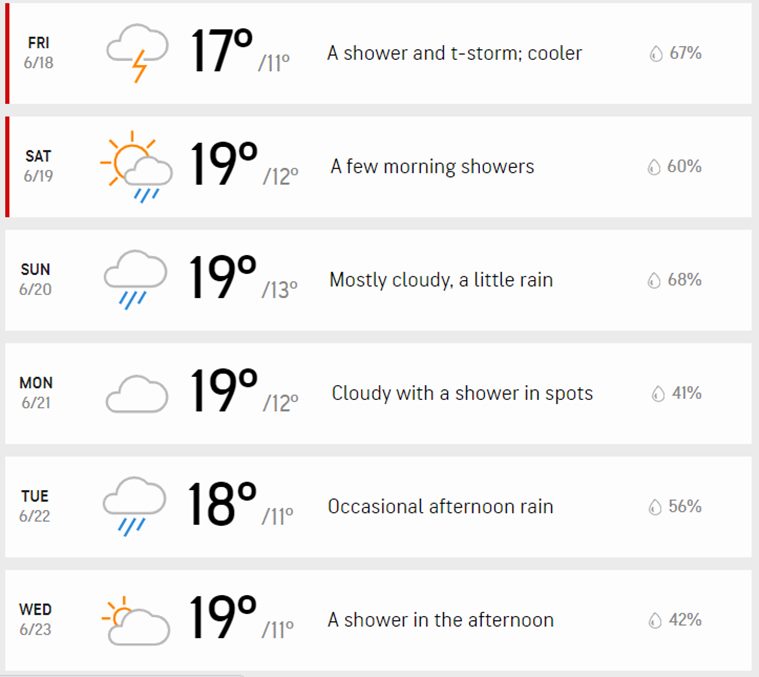A detailed weather forecast graphic is depicted in this image. The forecast spans across six days, starting from Friday and ending on Wednesday. The days are abbreviated in capital letters as FRI, SAT, SUN, MON, TUE, and WED. Each day is enclosed in its own rectangular segment within a long, horizontal rectangle that stretches across the entire image. 

Notably, the forecast for Friday and Saturday includes specific dates, 6-18 and 6-19, respectively. These days are highlighted with a vertical red line on the left side, possibly to emphasize the weekend.

For each day, the weather conditions are depicted through a small icon, followed by the high and low temperatures, described in degrees Celsius (e.g., 17°C/11°C for Friday). Further details include descriptive text about the weather and a percentage indicating the likelihood of precipitation. 

For instance, Friday's forecast shows an icon for thunderstorms, with temperatures listed as a high of 17°C and a low of 11°C. The accompanying text reads "A shower and thunderstorm, cooler," followed by a 67% chance of rain. The format and layout remain consistent throughout the rest of the days in the week, providing a clear and comprehensive look at the upcoming weather conditions.